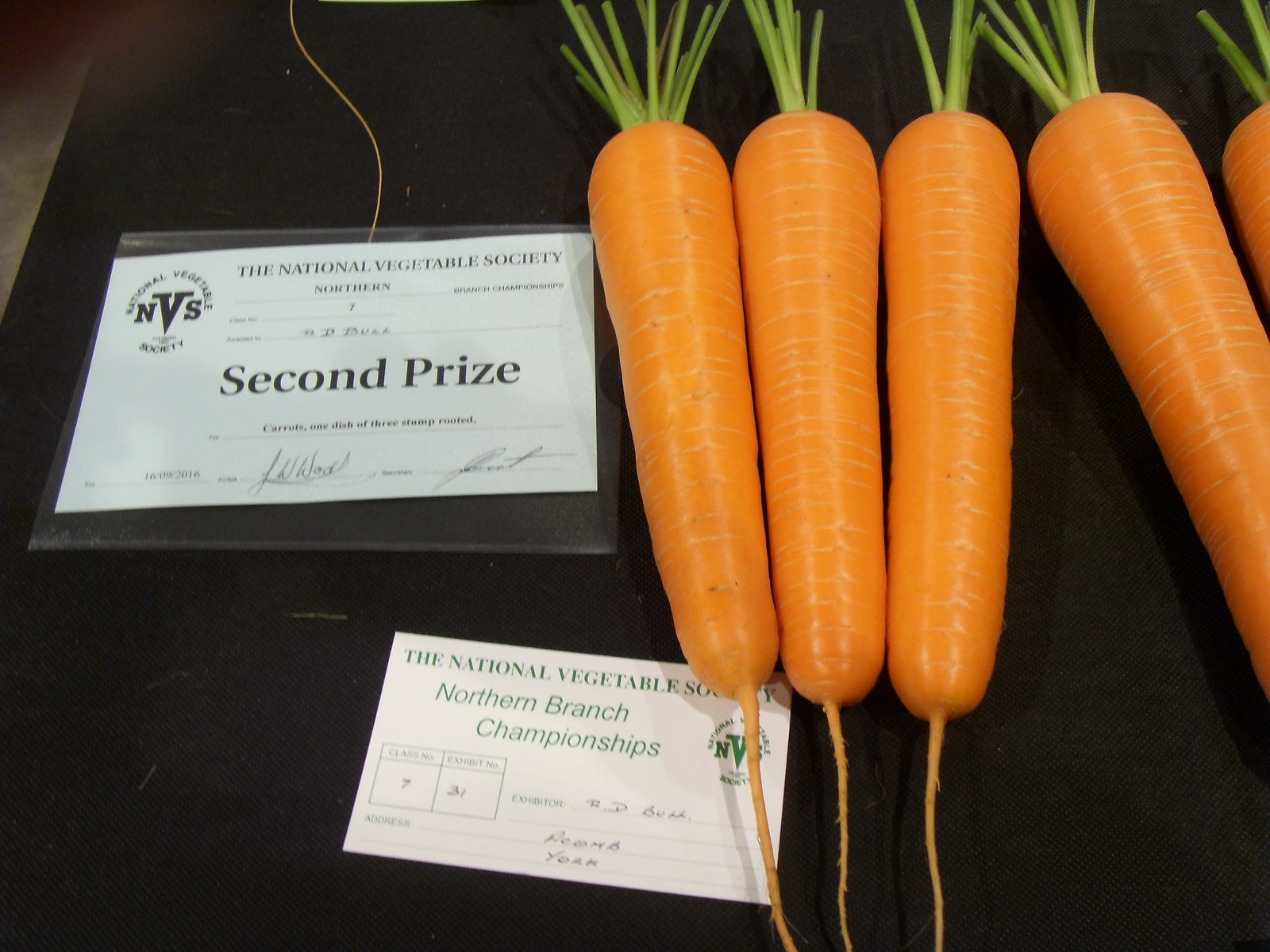On a black background, likely a tabletop, an assortment of objects is displayed. The focal point of the image is a collection of vibrant, orange carrots with lush green stems, each appearing exceptionally healthy and well-grown. To the left, a piece of paper prominently features "The National Vegetable Society" as the title. Below this heading, the text is too small to discern clearly in the photo. However, the visible portion confirms that these carrots have been awarded second prize by the National Vegetable Society. Beneath the carrots lies a card reading "The National Vegetable Society Northern Branch Championships," signifying the prestigious recognition these vegetables have received.